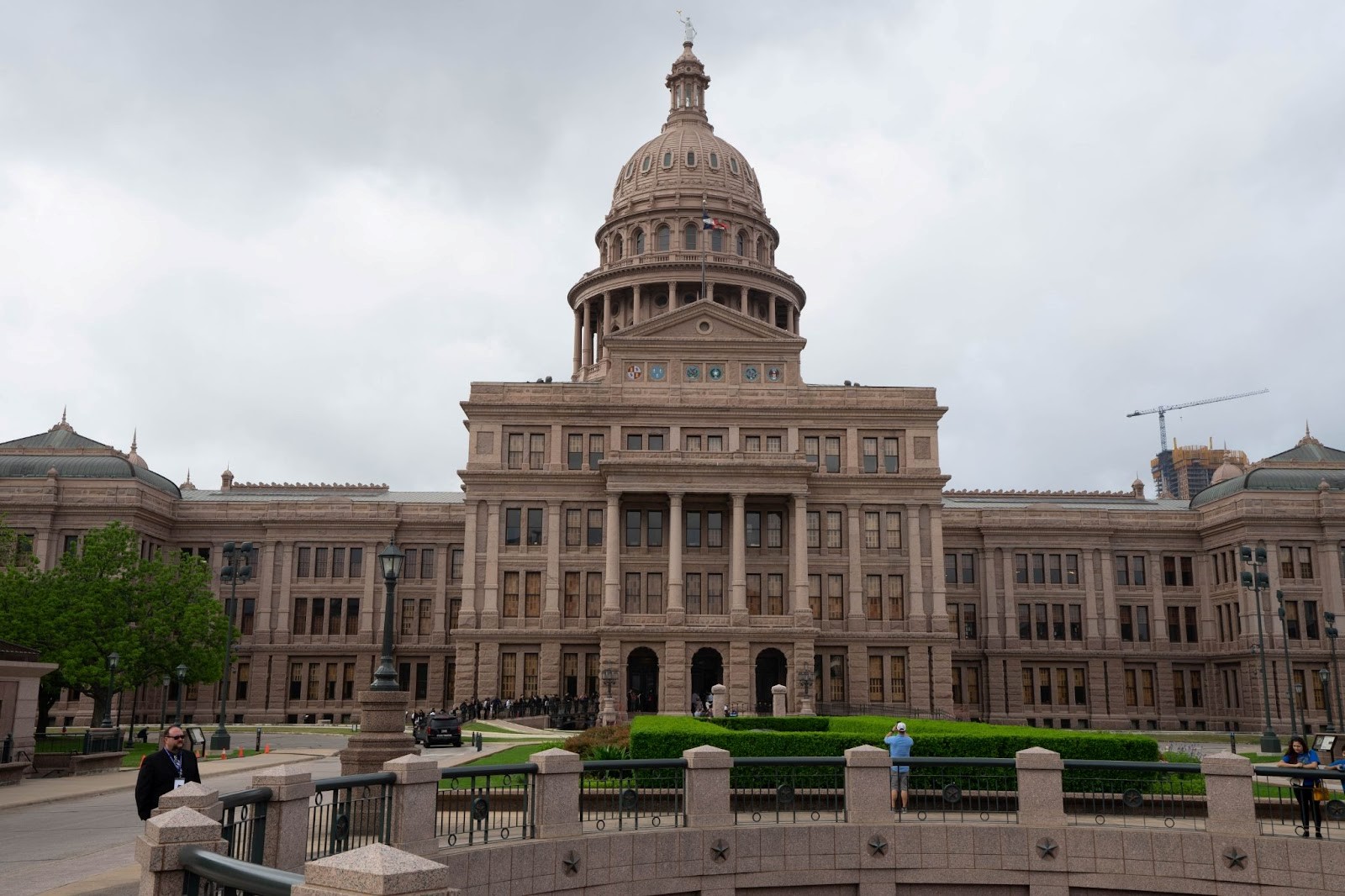The photograph captures a large, ornate building with a capitol-style dome at its center, crowned by a statue. Resembling a governmental or famous architectural structure, it features a central dome and ornate façade with four pillars and archways at the entry, flanked by east and west wings. The building's stone is a predominantly brown hue. In front of the building lies a courtyard with green grass and hedges, and several people are visible. On the left, a bald person wearing a black jacket and glasses stands, while to the right, a person in a blue shirt is visible. Central to the scene, another individual in a blue t-shirt, shorts, and a white baseball cap appears to be taking a photo of the building. The left side of the image also shows a tree with green leaves. In the foreground, a fence or wall suggests the presence of a freeway running underneath the area. Additionally, cranes can be seen to the right, possibly engaged in construction work on a rooftop structure.